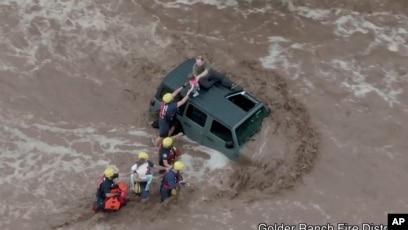The photograph vividly captures the tense, dynamic scene of a water rescue operation amidst muddy, churning floodwaters. At the center of the image is a dark green SUV, partially submerged and surrounded by the swift current. Two individuals—a child and an adult—are perched precariously on its roof. Five rescue workers, all wearing yellow helmets, are battling their way through the turbulent water towards the vehicle. The first responder has already reached the SUV and is extending a hand to the child. Another responder, distinguished by an orange bag, is amongst the group, suggesting coordination and preparedness. Various colors are noticeable in the image: the brown and gray hues of the floodwater, the green of the SUV, and the bright yellow helmets of the rescuers contrasted by their different colored tops. The photo is credited to the Associated Press, with visible text indicating "Golden Ranch Fire District," emphasizing the collaborative effort of first responders in a high-stress, urgent rescue mission.